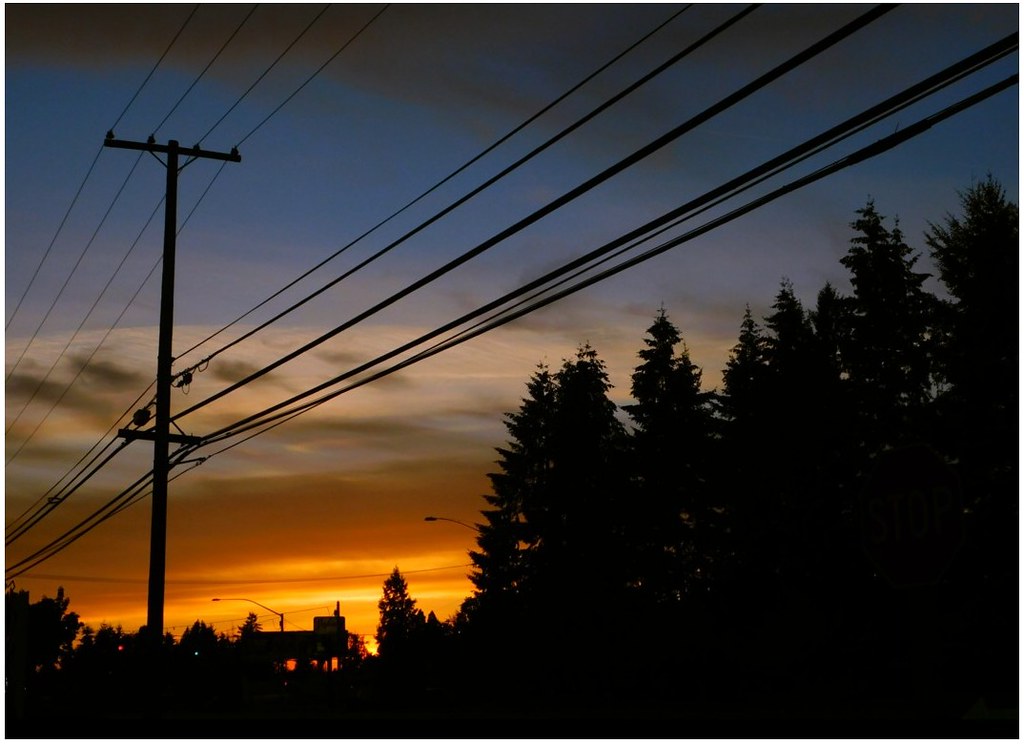This wide-angled photograph captures the serene transition of a day into night, either at sunrise or sunset. The sky displays a breathtaking gradient, transitioning from a deep blue with scattered clouds at the top to a glowing orange near the horizon. Dominating the top left section is a prominent telephone pole connected to multiple power lines, which stretch diagonally across the image from the bottom left to the top right. In the bottom right corner, a descending line of silhouetted conifer trees gently slopes down towards a building and a couple of unlit streetlights, located at the bottom left. These trees take up about three-quarters of the right side of the image. The mostly silhouetted scene creates a peaceful ambiance, accentuated by the last vestiges of sunlight illuminating the horizon behind the building, hinting it could be an industrial or business structure rather than a home.